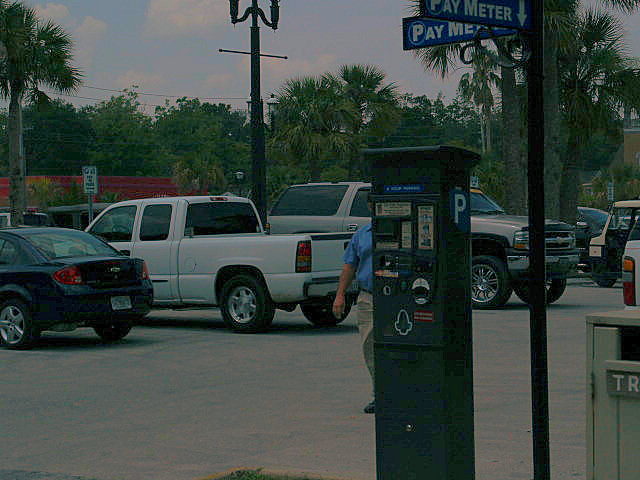In front of me is a dimly lit photograph capturing a bustling parking lot within what appears to be an American city. The image foreground highlights a green pay meter adorned with the words "Pay Meter" in white text on a blue sign, with an arrow pointing downwards. This pay meter partially obscures a man walking behind it, who is dressed in a blue short-sleeved shirt and khaki pants—his face and left side of the body hidden.

Directly to the right of this meter, a trash can stands, adding context to the scene. The parking lot hosts a variety of modern cars, including a sedan, a pickup truck, and an SUV, with additional vehicles visible in the background though not distinctly identifiable. The area is lush with vegetation, featuring green trees and distinctive palm trees. Despite the overall dark and shadowy quality of the photograph, the details of the environment, including the well-populated greenery and diverse collection of parked cars, stand out prominently.